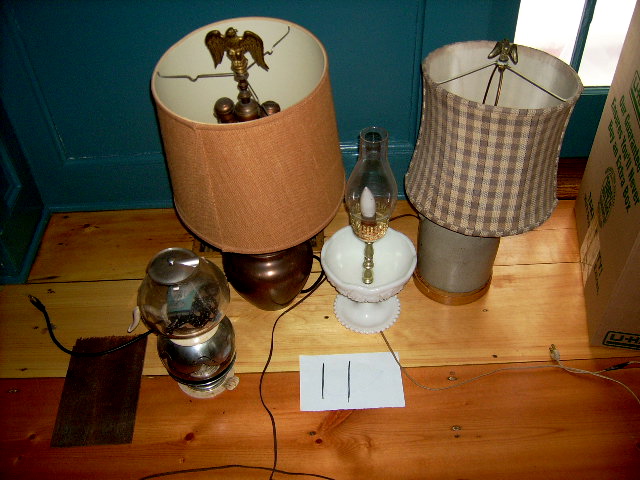This color photograph captures a cozy, somewhat chaotic scene of four distinctive lamps placed on a wide plank, light-colored wooden floor near a dark blue wall. These lamps appear to be staged perhaps as part of a moving process, evidenced by a large U-Haul mover’s box visible in the background. Natural light streams softly from a nearby window, illuminating the varied details of these lamps.

The first lamp on the left is minimalistic, featuring two small crystal orbs stacked on top of each other. Adjacent to it, the second lamp stands out with its white urn-shaped base and a small glass container at the top containing a single visible light bulb, lacking a shade. The third lamp is distinguished by its substantial gray body with a wooden base and adorned with a gray checkerboard lampshade, secured by a small eagle medallion. The fourth and final lamp, positioned to the right, stands tallest, with a bronze metal body and a tan cylindrical shade, also topped with an eagle medallion similar to the third lamp.

Together, these lamps create an eclectic ensemble, against the polished backdrop of the wooden flooring and the deep blue wall, capturing the essence of a transitional moment perhaps amidst a move.